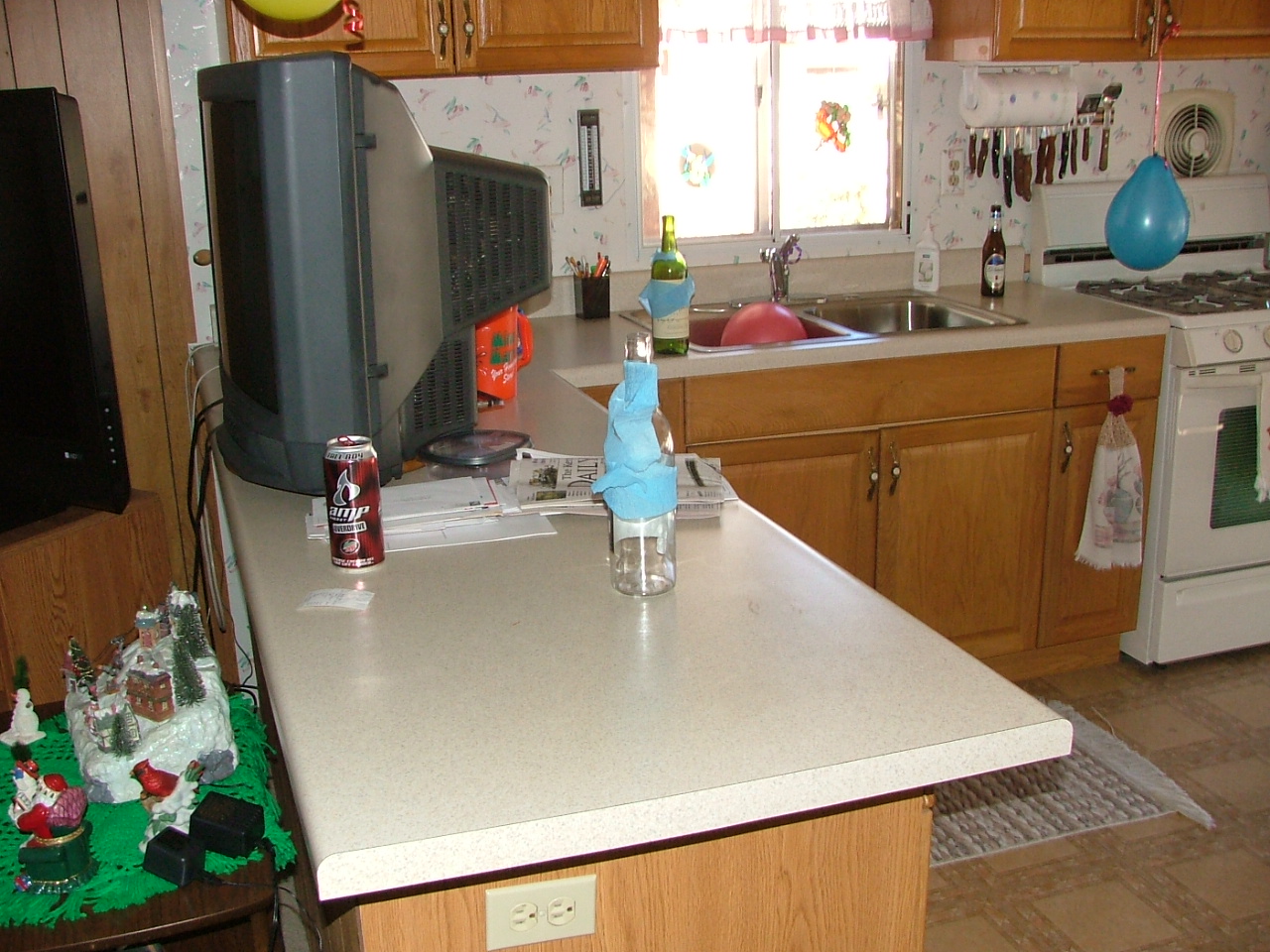Photograph of a cozy, well-used kitchen. The space features upper and lower brown wooden cabinets, complemented by a white speckled laminate countertop. Prominently, a stainless steel sink is situated in front of a window that bathes the room in daylight. On the right side of the kitchen, there is a gas stove, while on the left, an old-fashioned television faces a room adorned with wood paneling; its cords hang down noticeably. Evidence of a recent celebration is scattered throughout the scene. To the left, a small table displays figurines and a charming Christmas village. On the countertop, there are various items including an empty liquor or wine bottle, a stack of mail with a newspaper on top, and another wine bottle placed next to the sink. Adding to the festive atmosphere, a balloon sits in one basin of the double sink, while a beer bottle occupies the other half. Another balloon hovers above the stove, contributing to the lively and celebratory mood of the space.